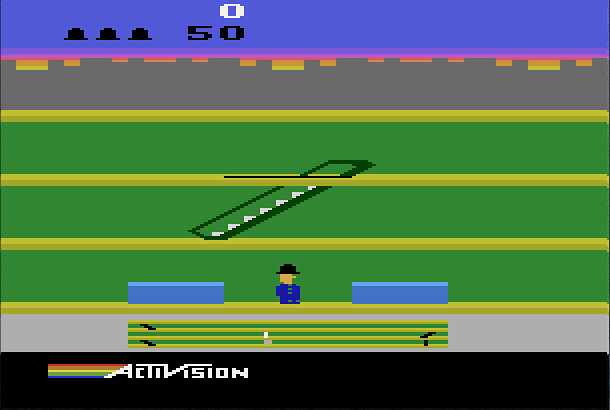The image depicts a screenshot from an old Activision game, likely from the Atari 2600 era. Dominating the top-left corner are three black objects resembling hats, alongside the number 50 in black with a white zero directly above it. The background features a simplistic, blocky blue skyline, framed by the outlines of buildings. The scene is divided into multiple layered sections colored with alternating bands of yellow and dark green. 

In the center of the image is a man clad in a blue coat and a black hat, standing between two blue rectangular blocks. This individual appears Caucasian with a tan pixelated face and is positioned at the bottom of the screen. A staircase in black with white steps is centrally outlined, connecting the first and second levels of the scene, enabling movement between these tiers.

Above the layered yellow and green bands, a grey area adorned with brown and yellow nodules is present, hinting at structural details. Below the man at the very base of the screen, fine lines in yellow and green create a rectangular pattern, bordered by small black segments. The picture is framed at the bottom by a broad black band featuring the word "Activision" in white, accompanied by a vibrant rainbow extending from the "A" and transitioning through red, orange, yellow, green, and blue colors.